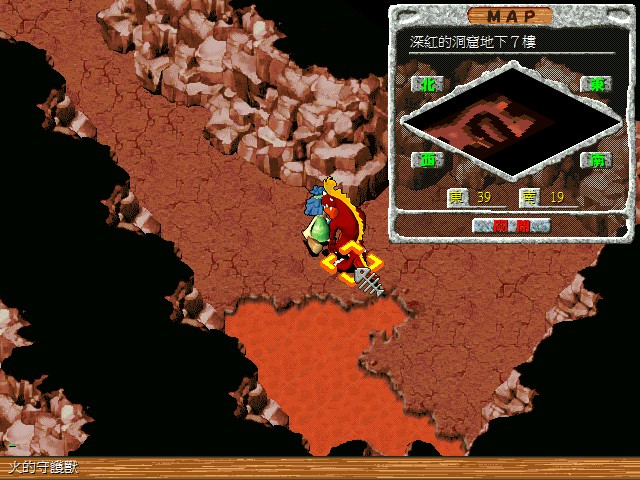The image is a detailed screenshot from an Asian-themed video game featuring a floating rocky and dirt platform against a predominantly black background. At the center of the scene is a red monster adorned with a distinctive yellow stripe running from the top of its head down its back. Surrounding the creature is a broken yellow box, and directly behind it, there is an icon depicting fish bones. The bottom right of the image fades into blank black space, while the bottom left reveals the jagged edges of another rocky platform. The top right corner of the screen contains a transparent map with a stone-colored border and Chinese characters on various icons. The word "map" can be seen at the top of this overlay. Additionally, there is a border at the bottom of the screenshot with wooden paneling and more white Asian text characters. The rocky surface of the platform includes piles of brown and orange elements that appear to be built up in places, resembling wood.